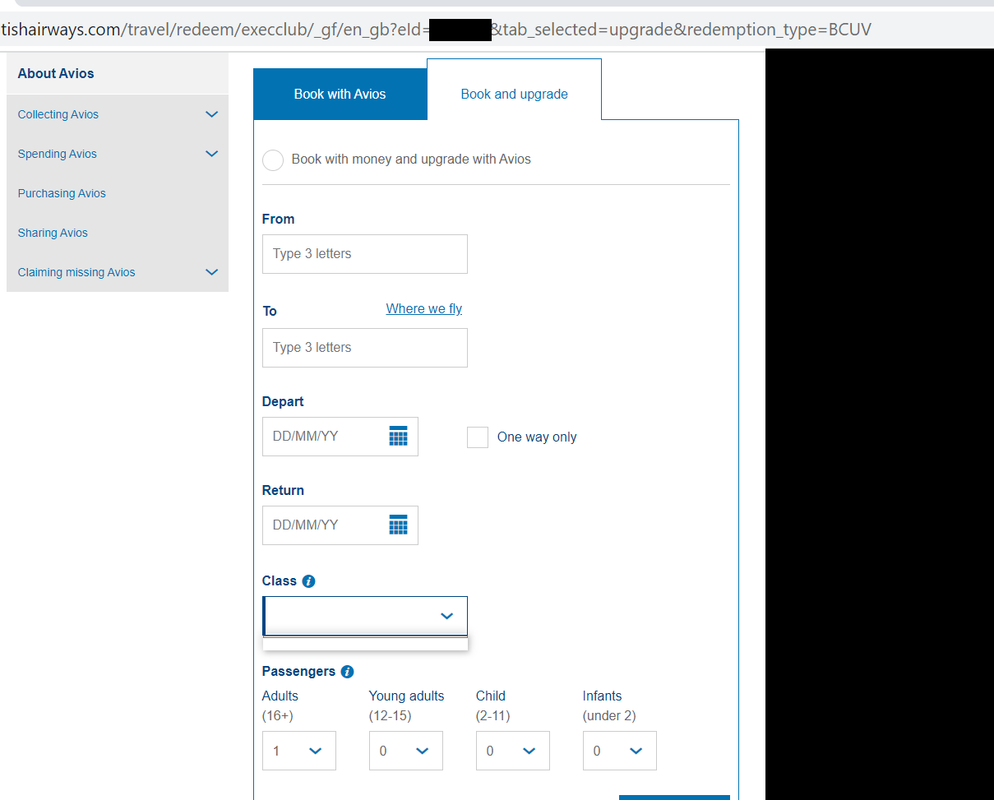This image displays a section of an airline's website, specifically the Avios program page. In the top-left corner, a navigation panel offers various options related to Avios, including "About Avios," "Collecting Avios," "Spending Avios," "Pricing Avios," "Sharing Avios," and "Claiming Missing Avios." On the right-hand side, there are two primary tabs: "Book with Avios" and "Book and Upgrade."

The screenshot focuses on the "Book and Upgrade" tab. Here, users have the option to "Book with Money and Upgrade with Avios." The interface includes fields for entering travel details, such as:

- **From:** A text box for the three-letter airport code of the departure location.
- **To:** A similar text box for the three-letter airport code of the destination.
- **Depart:** A date selector for the departure day, month, and year.
- **One Way Only:** A checkbox for one-way trips, ideal for those making a permanent move or who have no return plans.
- **Return:** A date selector for the return trip, if applicable.

Further options allow users to specify their travel preferences and details, including:
- **Class:** A dropdown menu to choose the travel class.
- **Passengers:** Fields to enter the number of passengers categorized as adults, young adults, children, and infants.

The interface is user-friendly and designed to help travelers easily book and manage their trips using Avios points.